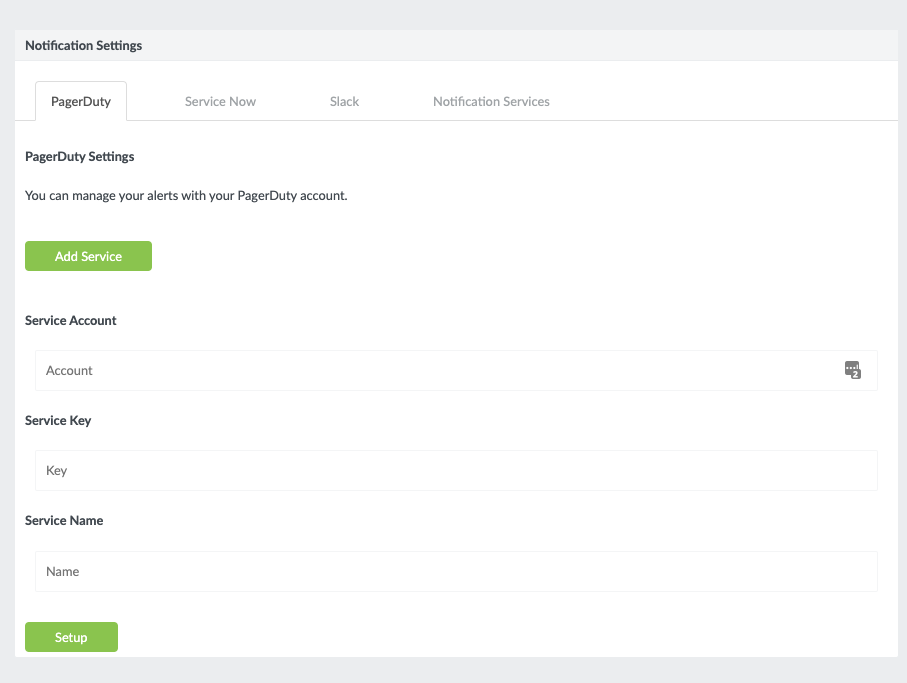**Caption:**

The screenshot captures a web-based form in landscape orientation, bordered by a gray frame, possibly indicating it has been placed on a gray card by the creator. The upper left corner of the form displays the heading "Notification Settings." Beneath this, a row of tabs spans from left to right, each representing a different notification service: PagerDuty, ServiceNow, Slack, and others. 

The current tab open is "PagerDuty," shifting the background to white for this section. The "PagerDuty Settings" heading is displayed prominently in black. Below this, an informative line reads, "You can manage your alerts with your PagerDuty account." A green button labeled "Add Service" follows.

Further down, the form fields require input for service configuration. The "Service Account" section has a field with a placeholder text "Account," next to a gray icon resembling a square with a number "2" in a smaller square overlaid. Following this is the "Service Key" section in bold, with a field labeled "Key." Finally, the "Service Name" section provides a field with the placeholder "Name."

In the bottom left corner, there's a noticeable green button with the text "Set Up" in white. This form allows users to set up and personalize their PagerDuty notification settings, adding and naming new services as needed.